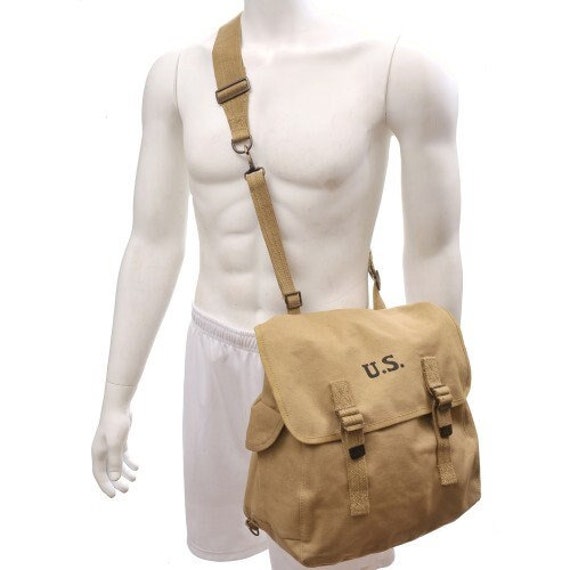This image displays the white torso of a headless mannequin, showcased from the knees up against a white background. The mannequin, clad only in a pair of white exercise shorts, prominently features a tan shoulder strap bag slung over its right shoulder and crossing its chest to the left side. This bag, which evokes the appearance of an old-fashioned U.S. mailbag, is emblazoned with the letters "U.S." on its overhanging flap. The knapsack-style bag also features two adjustable straps, likely for securing the front flap, and appears to have two pockets on either side. The overall visual impression is reminiscent of vintage army issue gear, possibly from the World War II era.